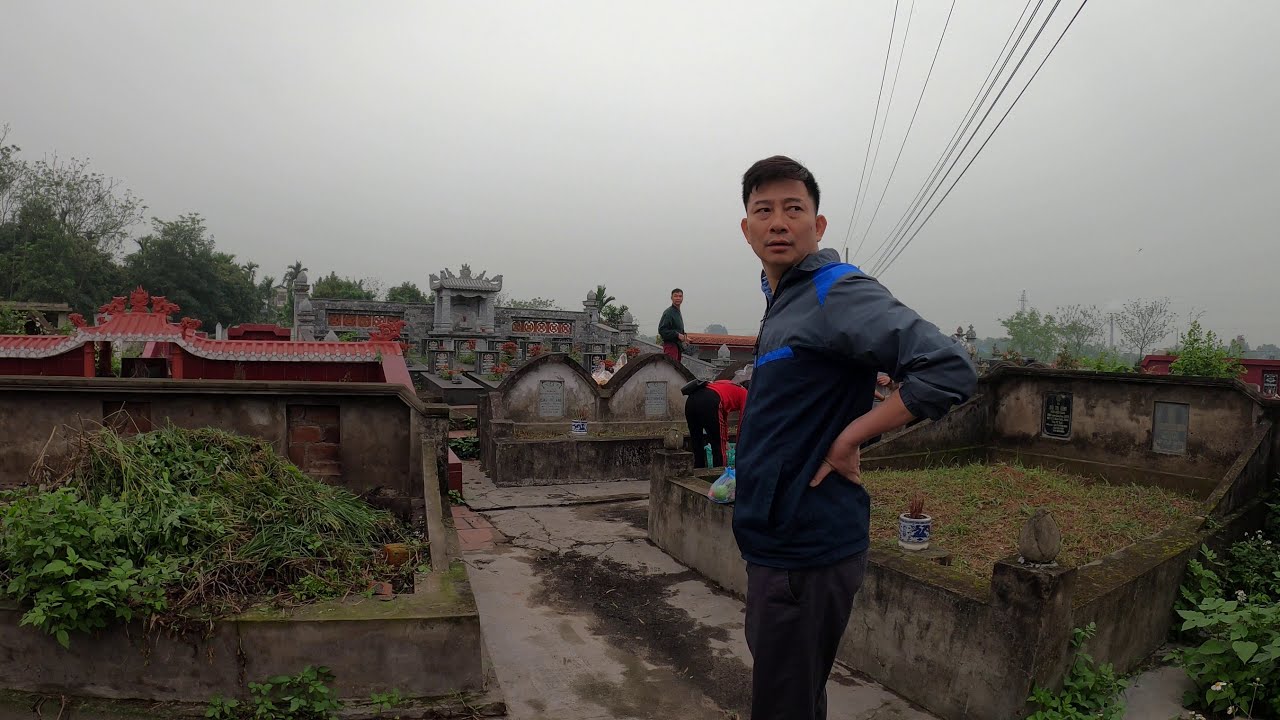In the image, an Asian man stands centrally with his hands on his hips, facing the camera. He is wearing a black jacket with blue accents and dark pants. His short brown hair catches the light under a gray, cloudy sky. The setting appears to be a rooftop filled with raised garden beds made of cement and concrete, flourishing with green grass and plants. Surrounding the man, several other individuals are engaged in tending to these gardens; one person, wearing a red and black outfit, is bent over their work, while another, clad in a green jacket and red pants, stands nearby. The backdrop includes distant buildings, green trees, power lines overhead, and structures resembling pillars or headstones, which contribute to the atmosphere of this urban, elevated garden space. The overall coloration of the scene leans towards gray and muted tones, with maroon elements adding subtle accents.